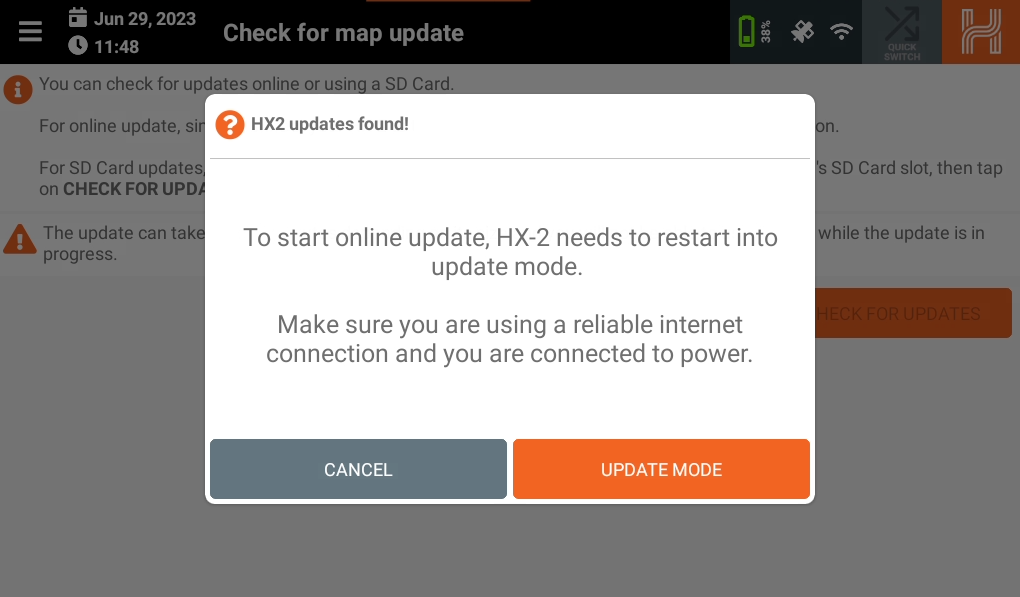Here’s a cleaned-up and descriptive caption for the image based on the provided information:

---

Screenshot of a webpage with a pop-up box obscuring parts of the content. The webpage features a light gray overlay and the top bar is black with a black border. On the top bar, from left to right, there's a hamburger menu, a date stamp "June 29th, 2023," a calendar icon, a clock icon with the time "11:48," and the text "Check for map update" in white. Further to the right, there are icons for battery status, sound, and WiFi connectivity. 

The page content includes a gray box and an orange box, with part of an orange "H" logo visible, composed of two squiggly lines forming an "H." Behind the gray overlay, there's an information icon with text stating, "You can check for updates online or using an SD card," although parts of this text are obscured by the pop-up box.

The white pop-up box contains an orange circle with a question mark on the extreme left. Text within the box states, "2 Updates Found!" followed by a line, and below it reads, "To start online update, XH-2 needs to restart into update mode. Make sure you're using a reliable internet connection and you are connected to power." At the bottom left of the pop-up box are two buttons: a gray "Cancel" button and an orange "Update" button. 

---